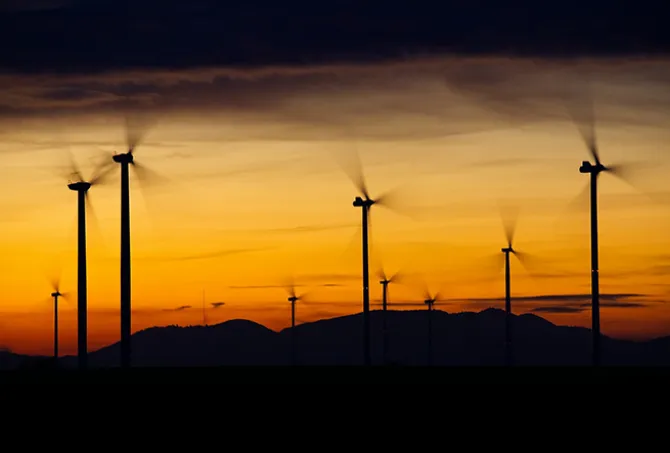This captivating outdoor image captures an evening sunset with a stunningly yellow sky. The upper portion of the sky transitions from dark, nearly black clouds, through shades of pink and dark purple, to white, and then becomes a wide strip of bright yellow before deepening into vivid orange closer to the horizon. Stretching across the photograph are rolling black hills, suggesting a silhouette of a mountain range. Dominating the landscape, a series of tall wind turbines spread from the left to right. The turbines, with their rapid, blurred three-bladed arms, stand prominently against the graduated hues of the sky, creating a mesmerizing blend of natural beauty and human engineering.